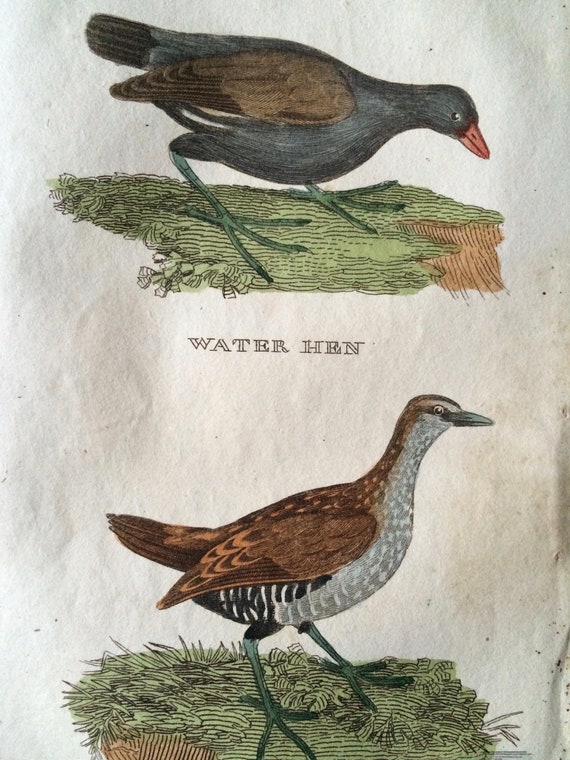The image depicts a detailed, classic drawing of two birds on worn, aged paper reminiscent of an old book. At the top, a blackbird with an orange beak and a single visible eye is crouched down with its head facing the ground. This bird has brown feathers on its wings and green talons. It stands on a patch of grass with dirt visible on the sides. Below the blackbird is the label "watcher" followed by another bird described as a "water hen." This bird stands upright on similar grassy ground, with its neck stretched out, showcasing a speckled grey breast and a brown back and wings. Its legs and beak have green hues, and the bird features black and white stripes near its lower body. The illustration, though not highly realistic, evokes a style akin to storybook art.